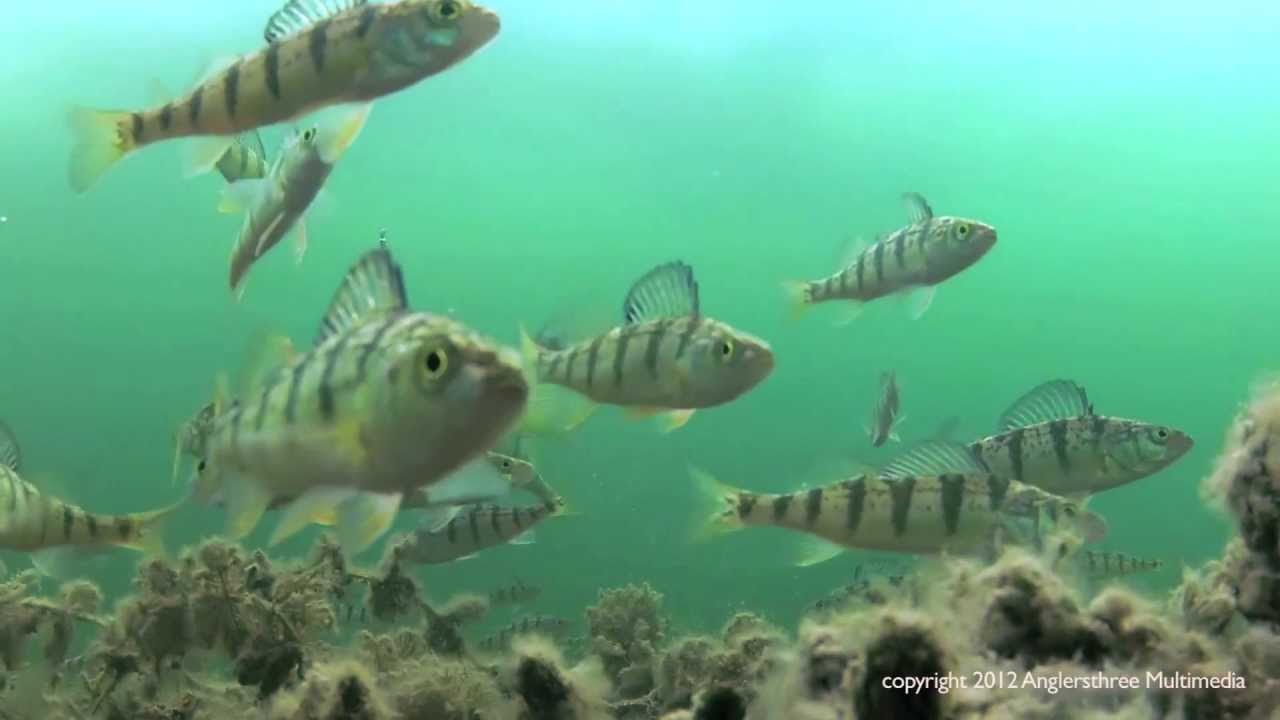This underwater color photograph, captured in a landscape orientation, showcases a small school of about 10 to 12 fish swimming in murky, turquoise-green water. The fish, which are beige to gray in color, feature distinctive vertical black stripes along their bodies. Each has a prominent, webbed dorsal fin that appears almost spiked, and sport large, round eyes with a golden hue. Near the bottom of the image, plant debris and coral-like structures resembling white and gray cotton balls line the lake or ocean floor. The scene is completed with a watermark in the lower right corner that reads "Copyright 2012, Anglers 3 Multimedia."